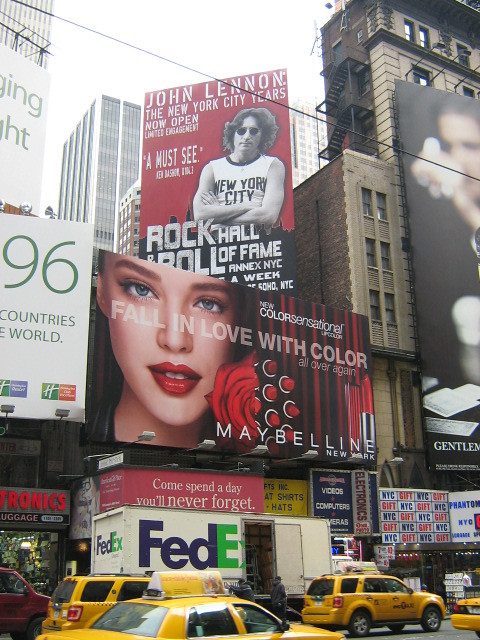In this outdoor image, the lower portion is dominated by vehicles, including four yellow cars and a dark red car at the bottom left. Behind the yellow cars, a white FedEx truck is visible, marked with the company's logo on both the side and back. The sky above the scene appears white. Positioned above the FedEx truck, a sign with a red background prominently displays the slogan, "Come spend a day you'll never forget," in white text. Further up, a larger billboard advertises Maybelline with the headline, "A new color, sensational lip color, fall in love with color all over again." However, the brand name is misspelled as "M-A-B-L-L-I-N-E."